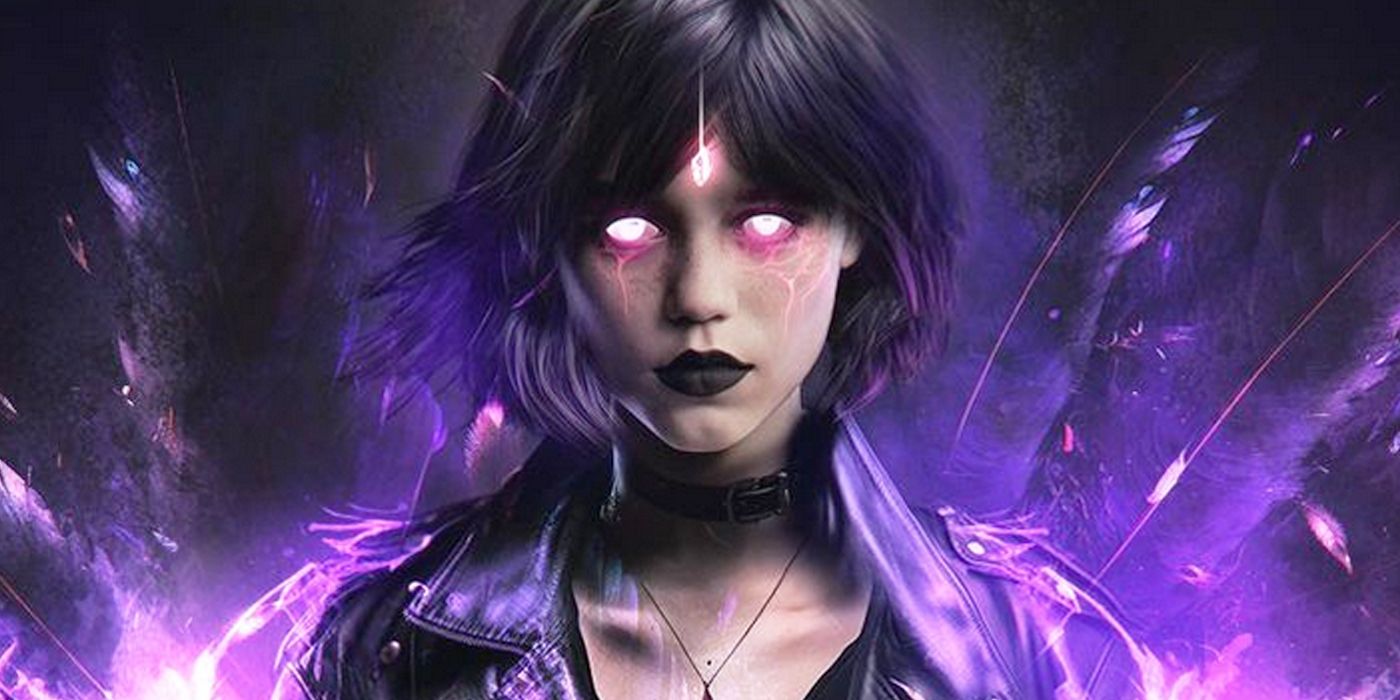This captivating illustration features a young girl adorned in a black leather jacket and a thick dog collar-style choker, complemented by a necklace. Her hair, which is short and black with wispy strands framing her face, is chin-length and transitions into ombre purple towards the ends. Her somber expression is highlighted by glowing eyes that appear to bleed pink tears, adding a striking and mysterious allure. Enhancing her gothic appearance, her lips are painted black and a radiant gem sits in the middle of her forehead, casting a light that splashes upwards. Purple lights, which fade into pink, emanate from her shoulders, creating a chaotic yet mesmerizing display of color that contrasts with the dark purple backdrop. These lights resemble feathers or spikes, contributing to the surreal atmosphere around her. Her pronounced collarbones give her a thin, almost ethereal appearance, emphasizing the delicate yet powerful visual elements. This haunting and vibrant imagery evokes a sense of otherworldliness, making her seem like a supernatural being, possibly a superhero or supervillain, bathed in an aura of shimmering lights.